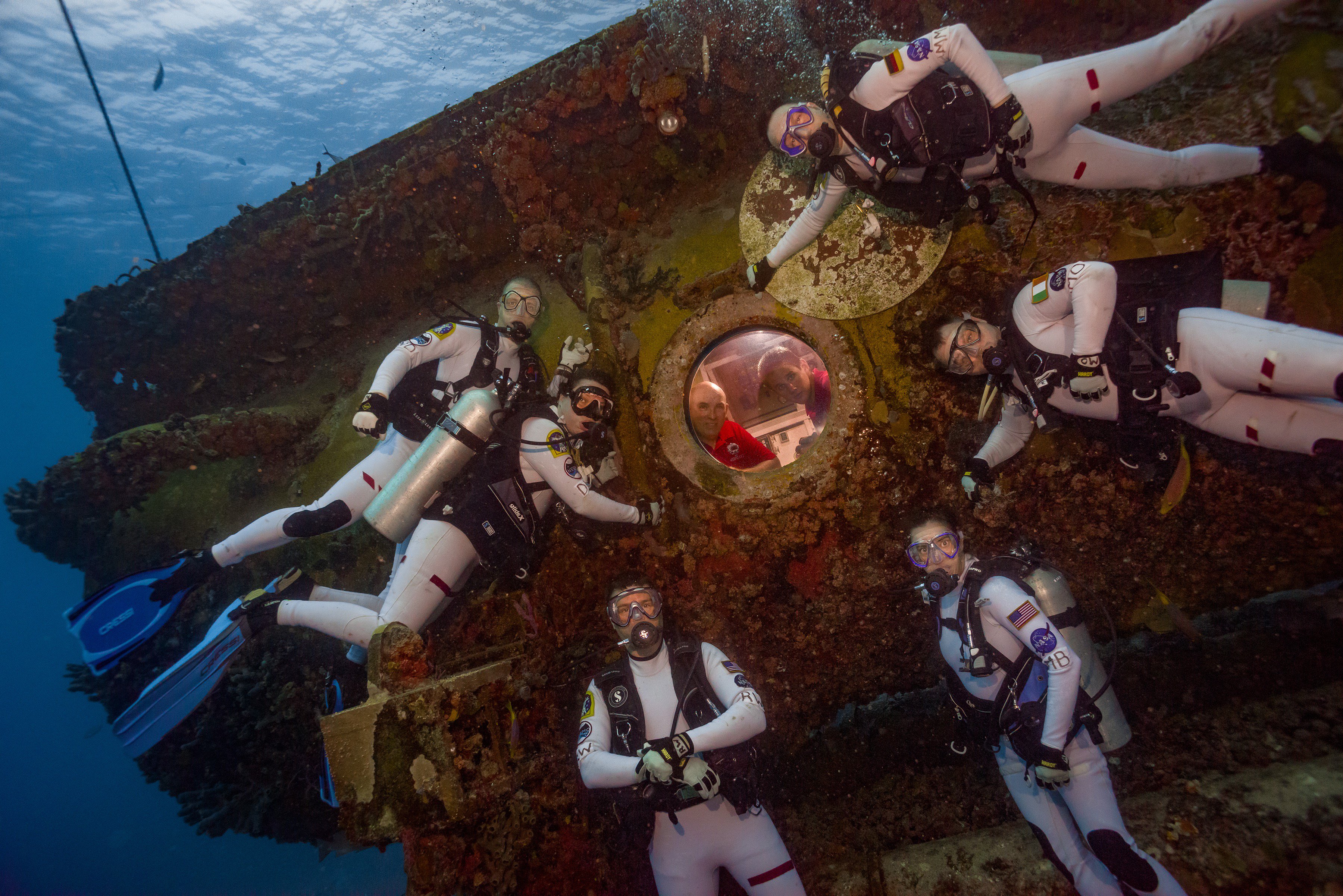This captivating underwater color photograph showcases a group of six divers posing around a yellow submersible, which is partially covered in rust, algae, and brown sea life. The divers, adorned in sleek gray wetsuits featuring national flags—American, Irish, and Spanish—are equipped with large silver oxygen canisters strapped to their backs via sturdy black harnesses. They sport blue swim fins and wear goggles with rebreather masks connected by tubes to their tanks. 

In the center of the image, the submersible's prominent round glass porthole draws attention, through which two individuals can be seen inside, dressed in distinct red shirts. One of the submersible's occupants is bald while the other has short brown hair. The interior of the submersible is illuminated, casting a soft glow on their faces as they gaze outward. 

The divers are intricately positioned around the submersible; one woman at the bottom displays an American flag on her shoulder, while nearby a male diver appears to recline against the submersible’s surface. Another diver clings to what seems to be a golden piece of the submersible at the top, having removed the porthole cover. The surroundings are perfectly framed by the ocean’s expanse seen in the upper and lower left-hand corners, adding depth to this fascinating underwater tableau.